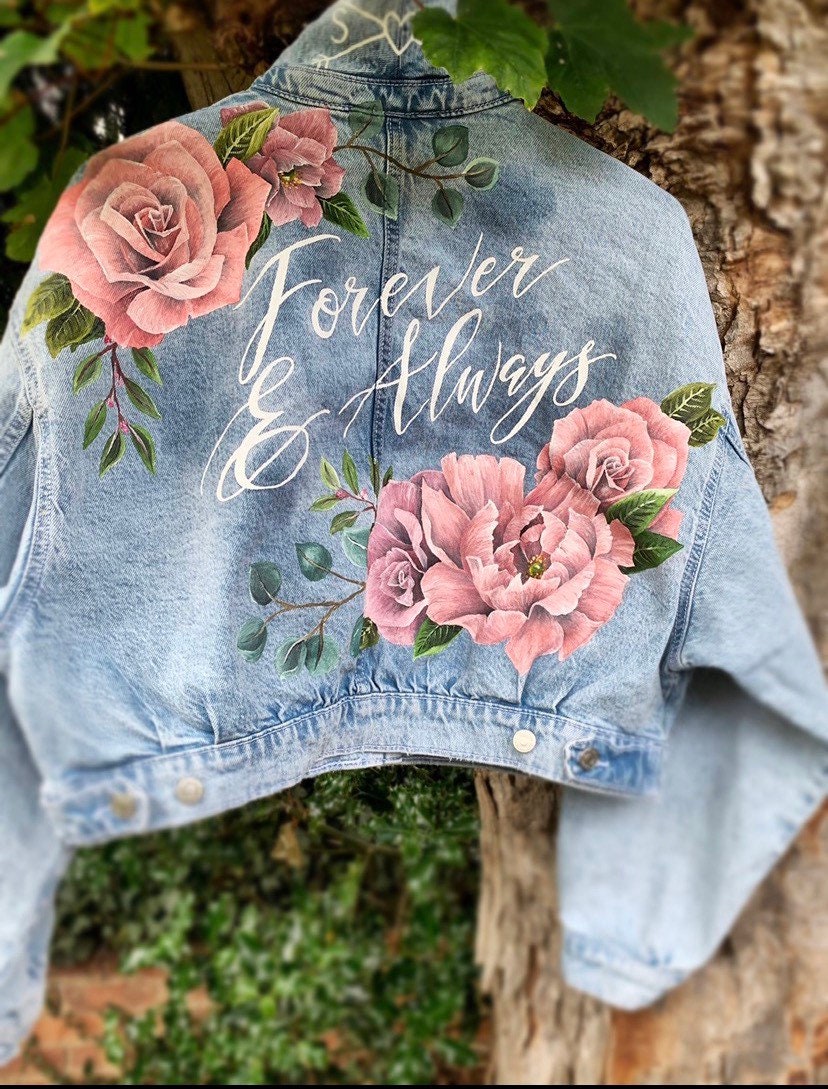The photograph captures a custom-decorated denim jacket hanging on a hanger from a tree limb, with a tree trunk visible on the right side of the image. The image, taken during the daytime, exclusively showcases the back of the jacket. The denim material features long sleeves and the torso part appears to be slightly cropped, possibly not covering the belly entirely. The jacket is adorned with vibrant, intricately designed rose motifs. On the upper left shoulder, there's a large pink rose with a smaller rose near the collar, both accompanied by branches and green leaves. On the lower right side, three similarly-sized roses, also with accompanying foliage, add to the aesthetic. At the center of the jacket, the phrase "Forever and Always" is handwritten or in a script-style font, with an upward incline to the right. Additionally, on the back of the collar, there is a heart with two arrows going through it, partially obscured by a leaf, revealing only the letter "S." The background shows leaves and vegetation, with some areas of the tree trunk intentionally blurred to enhance the jacket's prominence in the photograph.